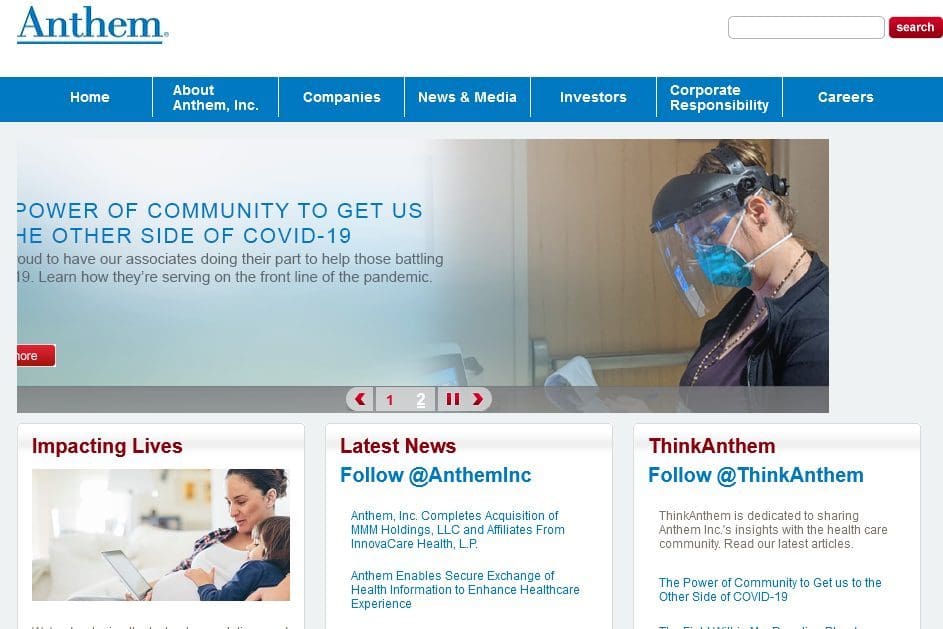In the top left corner of the image, the word "Anthem" is displayed in blue text. The top right features a white search bar with a red "Search" button.

Below this, there is a blue navigation bar containing several menu options: "Home," "About Anthem, Inc.," "Companies," "News and Media," "Investors," "Corporate Responsibility," and "Careers."

A prominent image dominates the lower section of the layout. It shows a woman wearing a heavy-duty black head shield with an integrated clear visor, a blue face mask, and blue goggles or glasses. She appears to be examining an item, possibly a bag, while standing in front of a door.

On the left side of this image, a headline partially reads, "Power of community to get us..." though the rest is cut off. Below this, more text is partially visible, discussing the efforts of associates in combating COVID-19: "Learn how they're serving on the front line of the pandemic."

At the bottom left, there is an image of a woman with her child, accompanied by the text "Impacting Lives." An adjacent box labeled "Latest News" encourages viewers to "Follow @AnthemInc." To the right of this, additional text prompts readers to "Think Anthem" and follow "@ThinkAnthem," with some further text beneath these prompts.